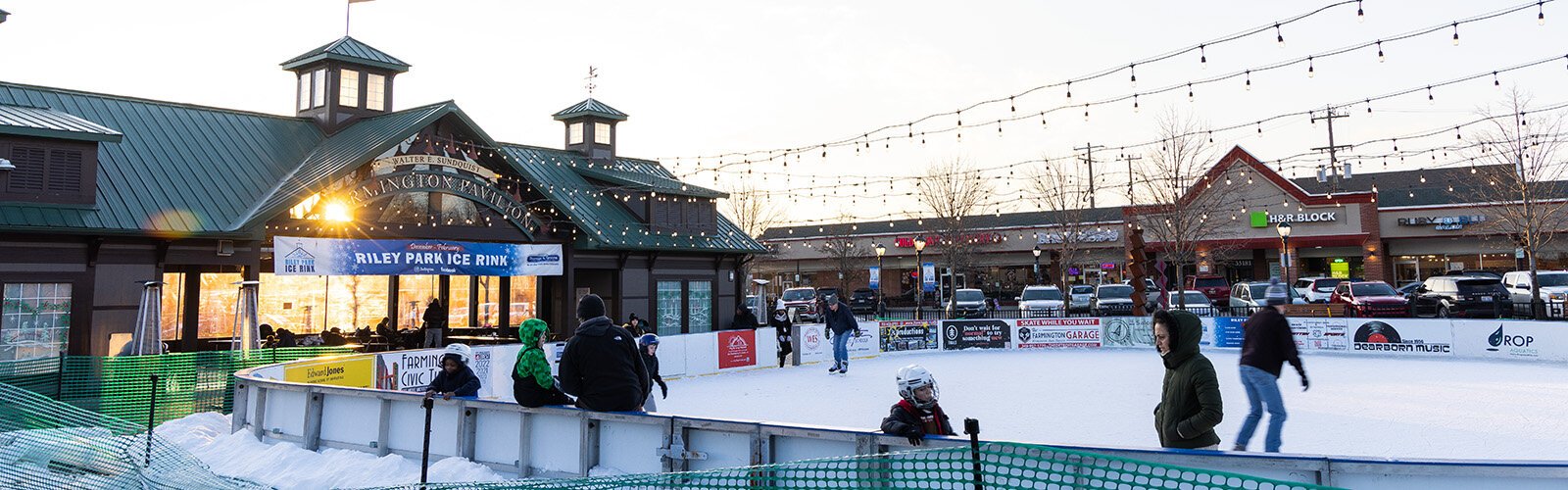In the winter scene depicted, an outdoor ice rink stands out as the main attraction. The rink is encircled by a white wooden fence adorned with advertisements on the inner walls, and string lights hang above, illuminating the area when it gets dark. Skaters gliding on the ice add life to the scene, framed by snow piled around the rink. A building adjacent to the rink, designated for the skating facility, boasts a dark green metal roof and windows that catch the sunlight. This building has greenish fencing around it and small, indiscernible signs. Beyond the ice rink, a business lot is visible with various establishments, though the only readable sign is for H&R Block. Numerous cars are parked in the lot, hinting at the area’s bustling activity. Flags flutter atop the building’s roof, adding a touch of color to the wintery tableau.